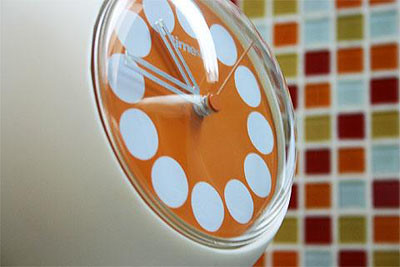The image depicts a vintage-style round clock, prominently centered and slightly tilted with its depth extending diagonally back to the left. The clock features a white plastic frame that partially disappears off the left edge of the image. The face of the clock is vibrant orange, adorned with twelve perfect white circular markers in place of numerical indicators. The clock hands are crafted from a shiny silver metal; both the hour and minute hands are uniquely hollow, forming squared ends. The second hand is slender and off-white. The hands indicate a time between 10 and 11, with the second hand pointing towards the middle left of the image. Just beneath the top white circle, the brand "Timex" is inscribed in white text.

The background features a grid-patterned wall composed of tiles in various colors including light blue, olive green, dark red, dark orange, and white, separated by white grid lines. This colorful tiled pattern enhances the overall vintage aesthetic of the scene.